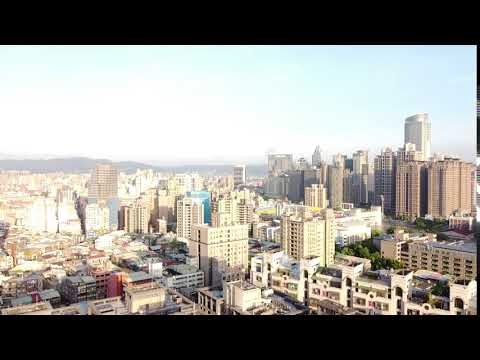This photograph captures a high-angle view of a sprawling cityscape taken from the top of a tall building. The image is framed by thick black horizontal borders at the top and bottom and thin vertical black lines on both sides. Dominating the lower right portion are white apartment buildings set against scattered trees, suggesting a small park or green central area. Progressing towards the center, the city features mid-sized white buildings transitioning to taller structures. The upper right section reveals clusters of brown office buildings dominated by a lone skyscraper that pierces the skyline. Further back, the cityscape culminates in an array of skyscrapers, with the buildings gradually decreasing in height towards the left, interspersed with slightly smaller skyscrapers. The horizon is defined by a distant mountain range beneath a light blue sky fading to bright white near the peaks.